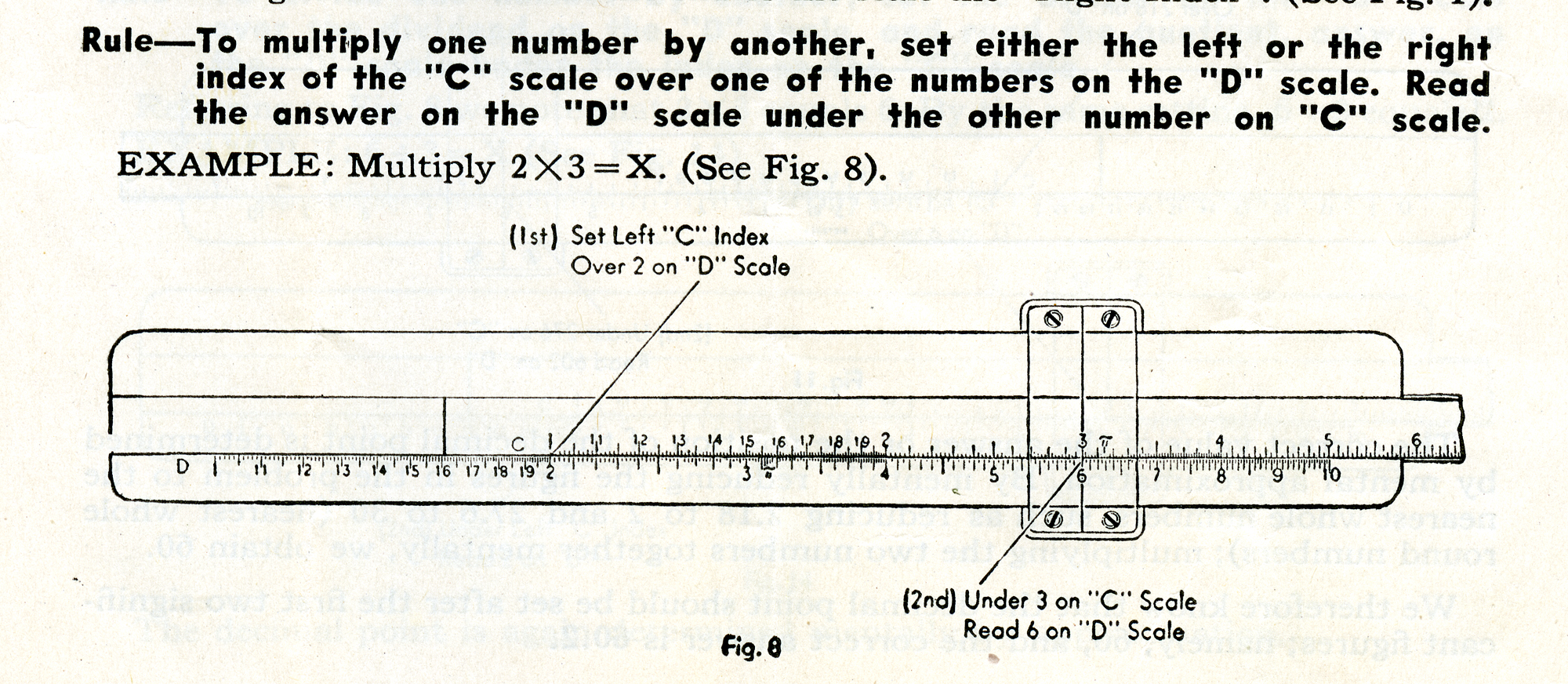This black and white diagram, likely from an older book, illustrates how to use a slide rule, a historical mathematical instrument. The page, appearing off-white with text faintly visible from the other side, features detailed instructions. At the top, it reads: "Rule: To multiply one number by another, set either the left or right index of the C scale over one of the numbers on the D scale. Read the answer on the D scale under the other number on the C scale." Below, an example states: "Multiply 2 by 3 equals X. See Figure 8." The illustrated slide rule shows the process: first, setting the left C index over 2 on the D scale, and second, reading the number 6 on the D scale under the number 3 on the C scale. The D scale displays numbers 11 to 19, and 2, while the C scale above starts at 1 and increments to 6. The bottom of the image is labeled "Figure 8", indicating its reference in the text.